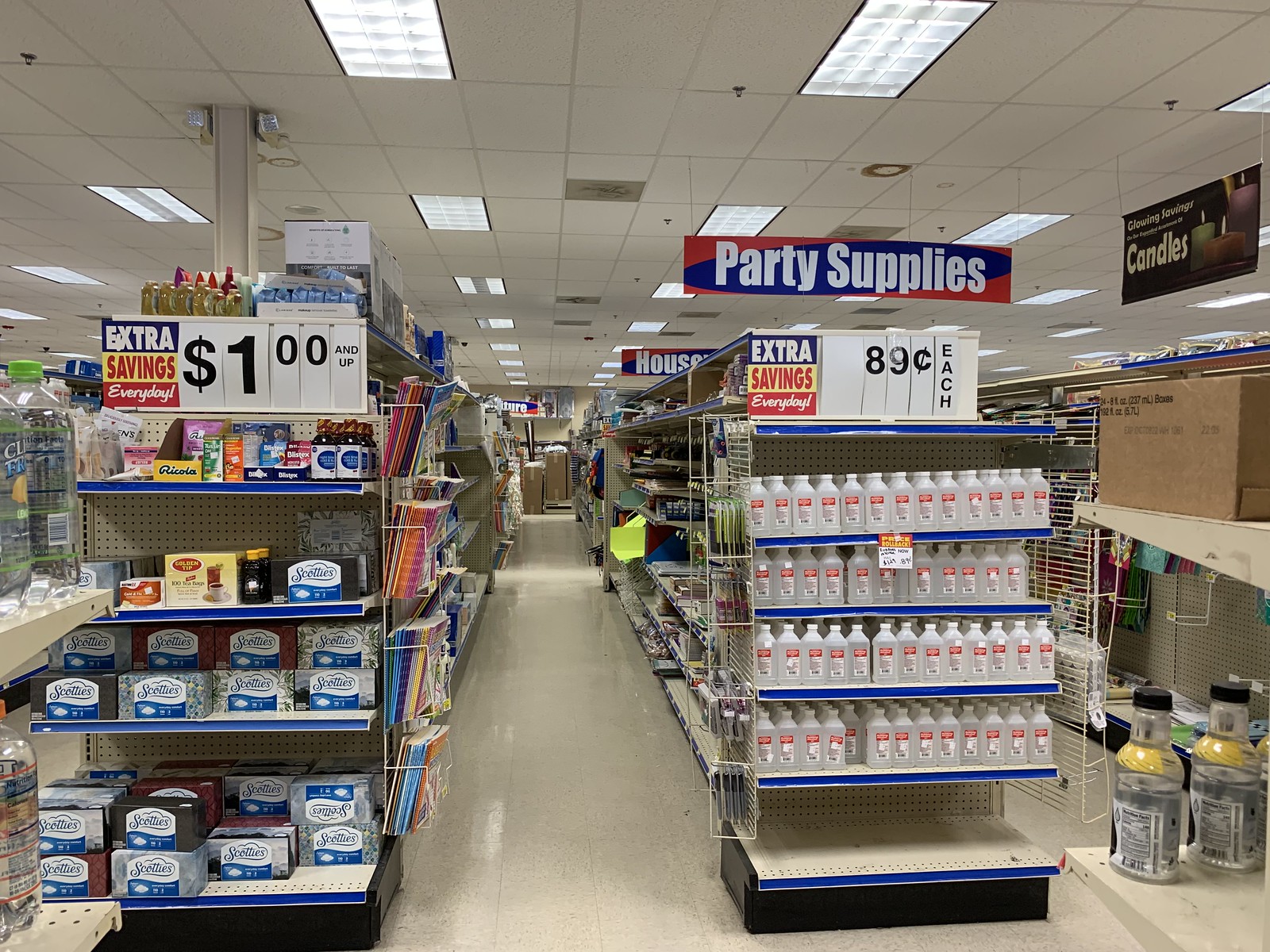This color photo captures the interior of what appears to be a dollar store, characterized by its long, narrow aisles lined with metal shelving. Prominent in the image, there is a sign overhead that reads "Party Supplies" in a red, white, and blue color scheme with a white font and a red and blue background. The shelves directly facing the viewer display a wide array of products, with the right-hand shelf featuring a sign that reads "89 cents each" and a display of white plastic bottles containing an unspecified liquid, possibly bleach cleaner. Adjacent to this, the left-hand shelf hosts box tissues with a $1.00 price sign above. Additional signage throughout the aisles promotes "extra savings every day" and mentions items priced "a dollar and up." In the background, various household items populate the shelves, and a sign indicating "candles" is visible on the right side of the image. The store's ceiling features visible tiles with embedded lighting, and notably, the aisles are devoid of people, accentuating the store’s quiet and unbusy atmosphere.